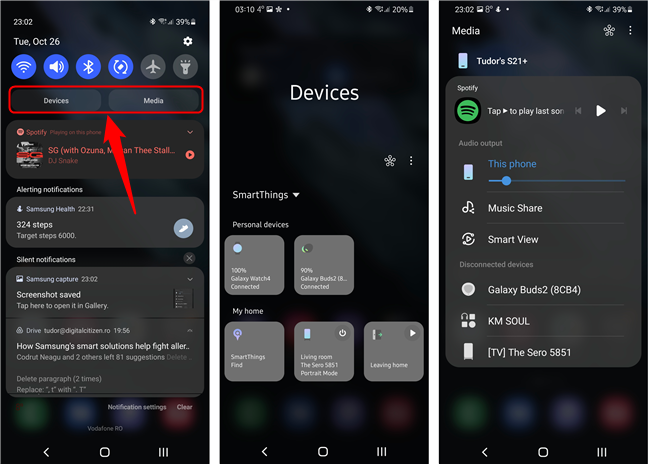The image showcases three smartphone screens displayed side-by-side, each presenting a different interface of the same device.

1. **Left Smartphone Screen:**
   - **Date and Time:** The screen displays "Tuesday, October 26th" at the top.
   - **Icons Row:** Below the date, there is a row of six icons:
     - **Grayed Out Icons:** Airplane mode and an unidentified icon.
     - **Active Icons:** Wi-Fi, speaker, Bluetooth, and screen rotation, all highlighted in blue, indicating they are turned on.
   - **Devices and Mode Section:** Below the icons row, a section labeled "Devices" and "Mode" is highlighted with a thick red rectangular outline.
   - **Red Arrow:** A prominent red arrow overlays the screen, pointing toward the "Devices" and "Mode" section, occupying about a third of the screen space.
   - **Text Boxes:** There are four gray text boxes with white lettering scattered across the screen, partially obscured by the red arrow. The background is slightly blurred, revealing app icons underneath.

2. **Middle Smartphone Screen:**
   - **Battery Status:** Displayed as "20%," indicating a low battery level, previously 39% on the left screen.
   - **"Devices" and "SmartThings":** The screen shows a section titled "Devices" and "SmartThings" (capitalized and merged together), with an expanded drop-down menu.
   - **SmartThings List:** Five gray squares are displayed:
     - **Top Row:** Titled "Personal Devices" with two gray squares.
     - **Bottom Row:** Labeled "My Home" with three gray squares, suggesting they are smart home devices, although the exact details are unclear.
   - **Background:** The interface is set against a black backdrop.

3. **Right Smartphone Screen:**
   - **Battery Status:** The battery level is at "39%," higher than the middle screen.
   - **Media Section:** 
     - **User Identification:** Named "Tudors S21" (not as a teacher but spelled "T-U-D-O-R-S").
     - **Spotify Interface:** A notification for Spotify indicates "Tap arrow to play last song" along with other audio options such as:
       - Audio input source: This phone
       - Music share
       - Smart view
       - Galaxy Buds 2
       - KM Soul
       - A TV
     - **Slider Bar:** A slider bar at the bottom, which likely controls volume or another adjustable setting.

The composition of the image is designed to provide an overview of different functionalities and configurations across the three screens of the smartphone.